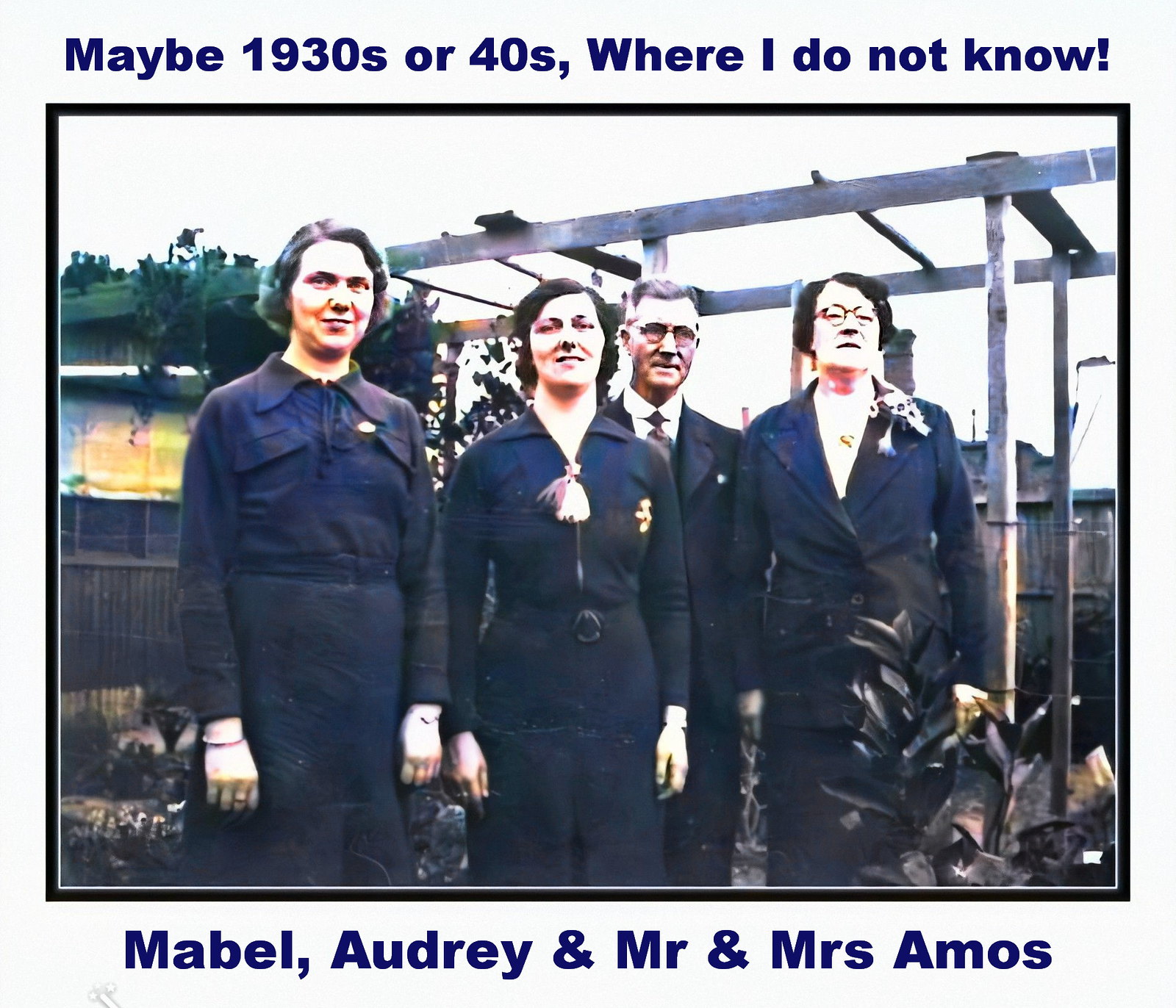A sepia-toned photograph seems to capture a mid-20th century gathering, possibly from the late 1950s or early 1960s. The image features names like Mabel Audrey and Mr. and Mrs. Amos, suggesting an older era. The setting appears to be a backyard, hinting at an informal event. The clothing styles, including a woman wearing pants, further indicate a time when such attire for women was becoming more socially acceptable. The photograph has a military touch, possibly a family reunion or a wedding, given the mixed formal and casual attire of the people.